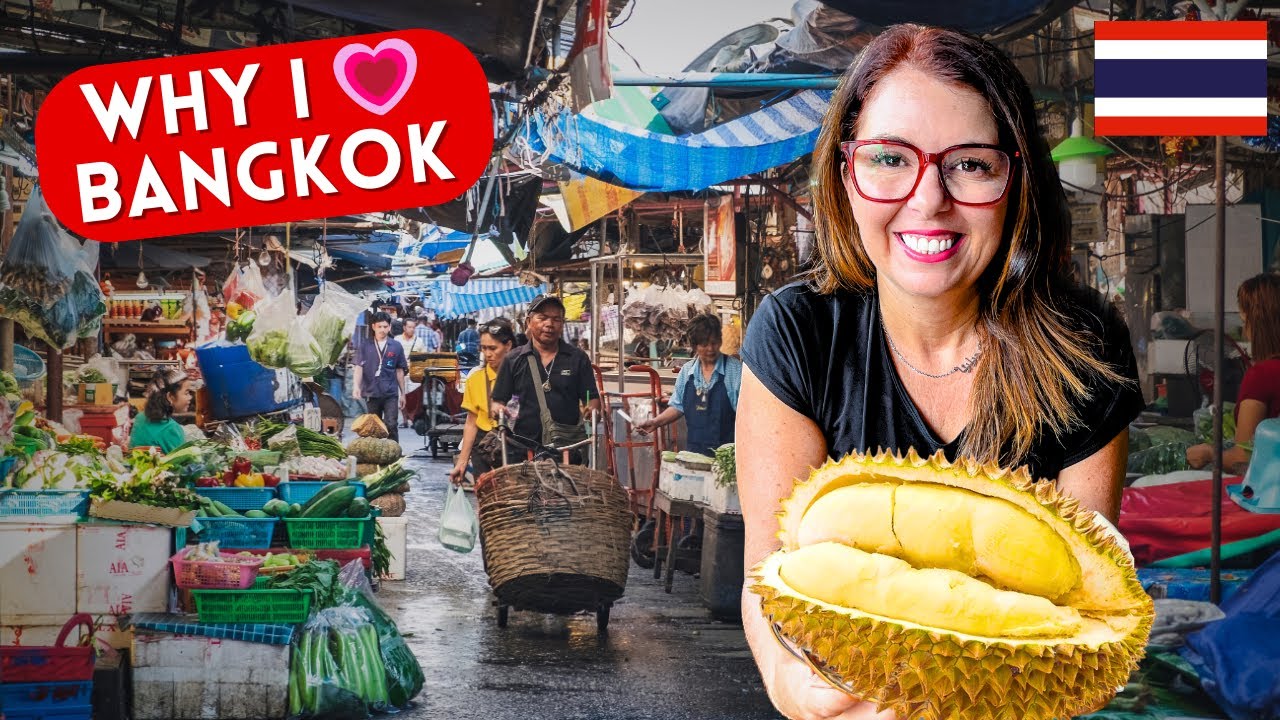This image, likely a YouTube video thumbnail, features a bustling marketplace in Bangkok. In the background, various stalls display fresh produce and goods, while people, including a man pushing a dolly with a large basket, engage in their shopping activities. Dominating the right side of the image is a smiling woman with shoulder-length brown hair wearing large, square red glasses and a black short-sleeved v-neck top. She is holding up a durian fruit, showcasing its spiky exterior and soft, yellow interior. In the top left corner, a rectangular banner reads "Why I ❤️ Bangkok," and the Thai flag is visible in the top right corner, hinting that the woman might be discussing her love for visiting or living in Thailand.